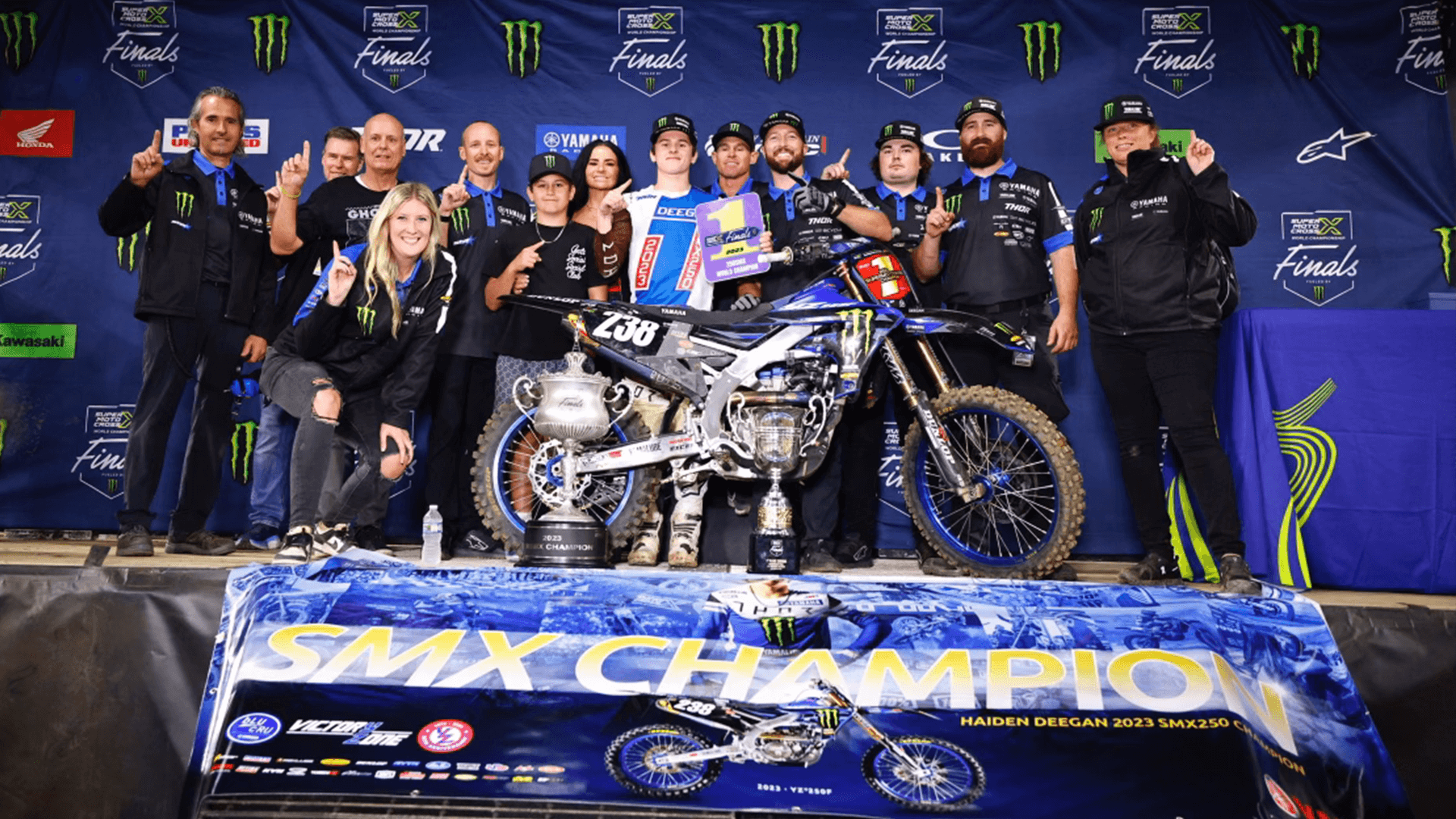The image depicts a lively trophy presentation at the 2023 SMX World Championship Final held at the LA Coliseum. Central to the scene is a blue BMX bike, emblazoned with the number 238, standing prominently on a podium. Flanking the bike are two large silver trophies, underscored by a banner that reads "SMX Champion." The backdrop features a large, colorful display promoting various sponsors, including Monster Energy and Yamaha. A jubilant group of 14 individuals, including the winning rider and team members, are assembled on stage, many sporting Monster Energy logos on their jackets and holding up their first fingers in a victory pose. The stage is vibrant with excitement, set against a blue-themed banner showcasing the bike and the championship's grand finale.